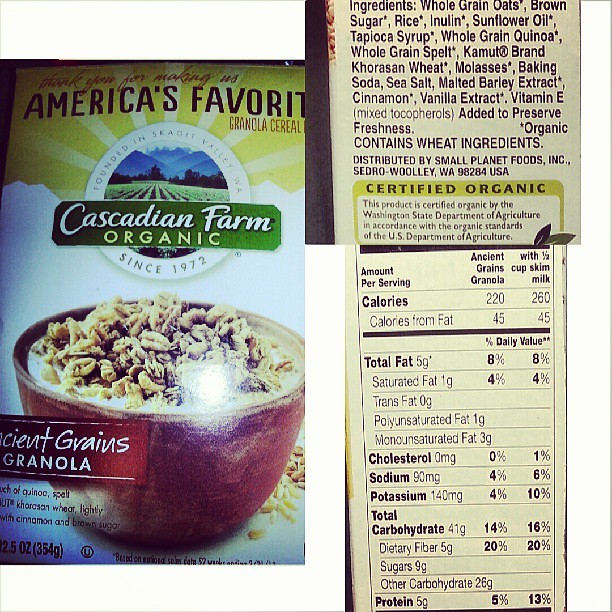In this vertically-oriented, slightly rectangular image frame, there are three distinct photographs presented. The left half of the frame prominently features the front of a cereal box, though the lower left portion of the box extends out of the frame. The top section of the box displays a cheerful yellow background with light beams representing a radiant sun. Just beneath, a green banner showcases the brand name, "Cascadian Farm Organic." Below the banner, there is a bowl of cereal depicted, crafted from a reddish clay or pottery material. Notably, the image has a flash glare that partially obscures the bowl. On the right side of the frame, two side labels are stacked vertically. The upper label details the ingredients list, while the lower label provides the nutritional information of the product.